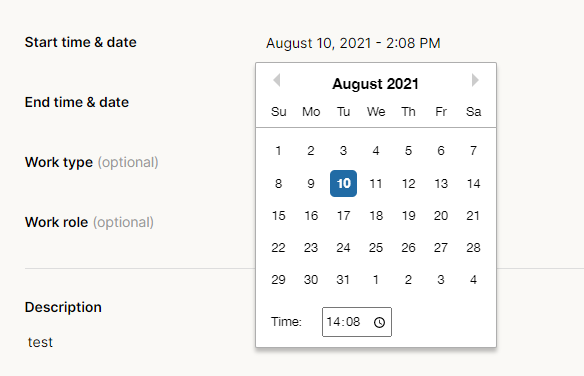A screenshot of a calendar application with an off-white to light gray background. The interface includes black text in the top left corner displaying "Start Time" and "Date," followed by "End Time" and "Date." Below these, it reads "Work Type" with the word "optional" in lighter gray parentheses, and then "Work Role," also marked as "optional" in lighter gray text. A horizontal line separates this section from the next. Beneath the line, the word "Description" appears in black text, followed by the word "test" in dark gray, all lowercase. The calendar is set to August 10, 2021, at 2:08 PM, highlighting Tuesday, August 10, and the time 14:08 on the accompanying monthly calendar view.